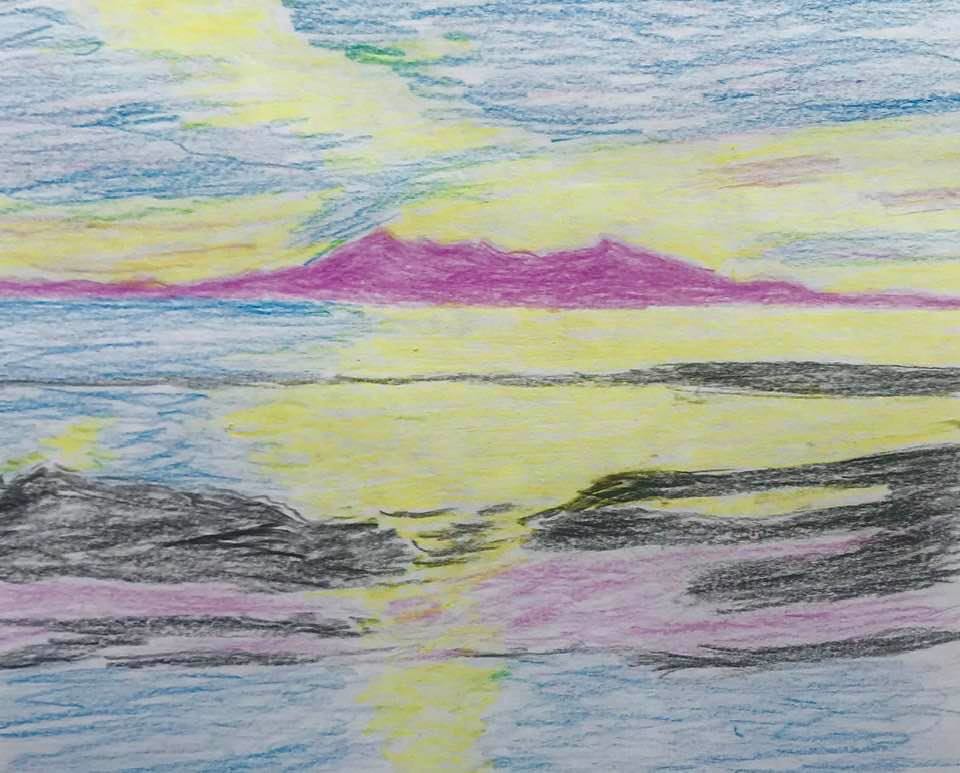This image features an expertly crafted drawing, likely created with crayons or pastels, showcasing an impressionistic sunset scene over water. The artwork, characterized by its abstract and evocative style, beautifully captures the essence and mood of the setting sun. The primary color of the water is a deep, calming blue, mirroring the clear blue sky above. The sun, depicted in a radiant yellow, glows vividly behind a wispy pink cloud, casting a warm hue across the horizon. In the distance, a hint of land or perhaps a jetty, rendered in a stark black, adds depth and contrast to the serene seascape. Despite the lack of fine details, the drawing's skilled execution conveys the tranquil and picturesque moment with remarkable clarity and beauty.